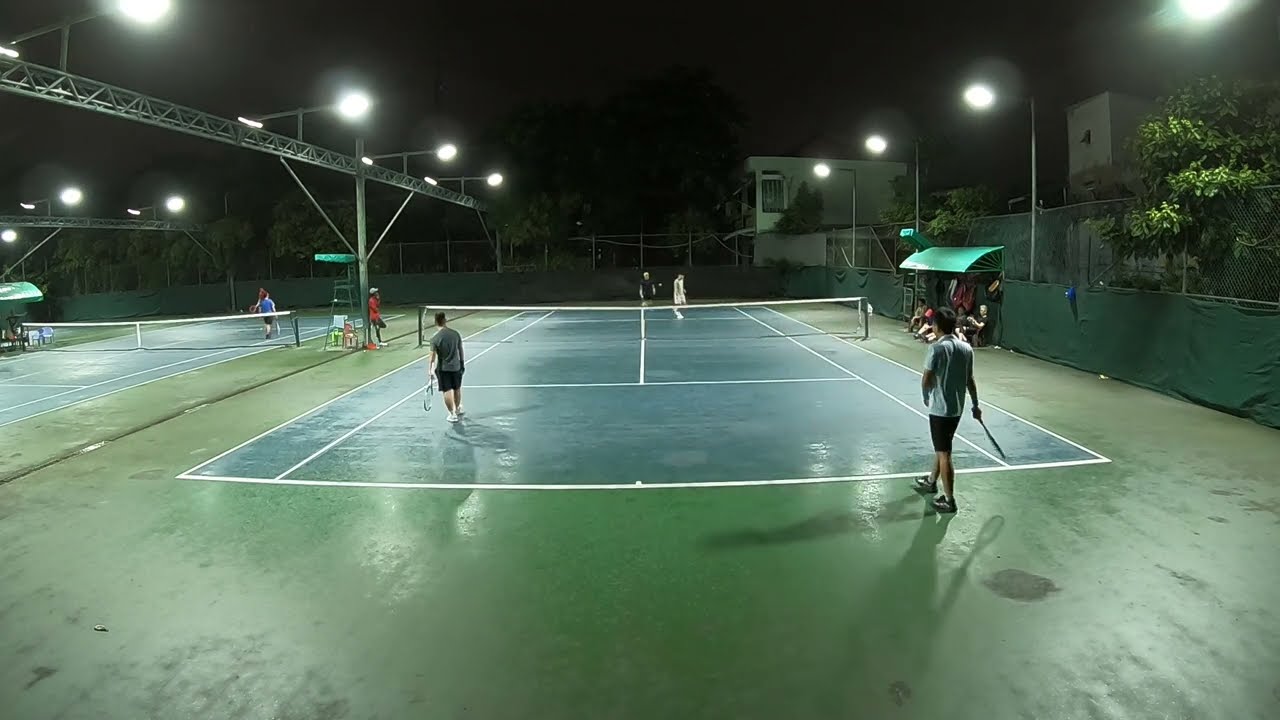This is a detailed nighttime photograph of an outdoor tennis complex featuring two tennis courts. The courts have a green surface with white boundary stripes and a vivid teal-blue playing area. They are illuminated by multiple light fixtures mounted on metal structures. The dark night sky contrasts with the bright lighting of the courts, where several players are engaged in a match. 

On one court, two players in gray shirts and black shorts compete against two opponents; one dressed in white, the other in black, possibly wearing a hat. There is another pair of players on the adjacent court. Both courts are enclosed by a chain-link fence, with lush green trees and residential buildings visible beyond the barriers.

Midcourt, a green awning provides shelter, possibly for observers or a referee, adding to the organized setting. The venue appears to be a public-use tennis facility within a city, potentially hosting a competition. The overall ambiance is vibrant, with the glowing lights and the dynamic activities of the players and spectators.